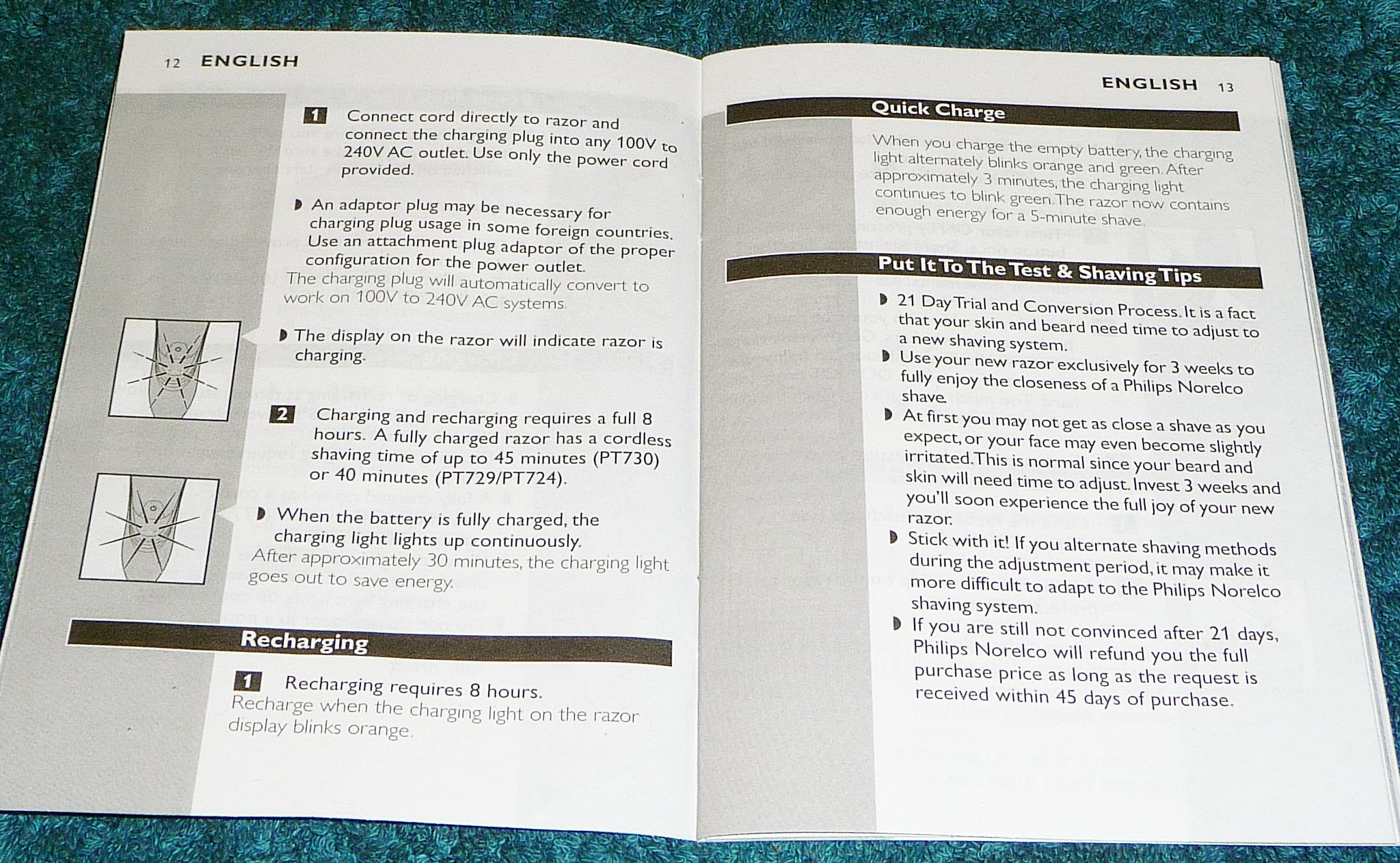This black and white photograph shows an open instruction manual, specifically pages 12 and 13, with details about a Philips Norelco razor. The page numbers are visible in the top corners: "12" on the upper left and "13" on the upper right, both accompanied by the word "English." 

Page 12 is dedicated to recharging instructions, starting with:
1. Connect the cord directly to the razor and use the provided power cord for any 100V to 240V AC outlet. An adapter may be needed in some countries. The charging plug adapts automatically to different voltage systems, and the razor’s display will indicate it's charging.
2. Charging takes a full 8 hours, providing up to 45 minutes of cordless shaving. A charging light displays continuously when the razor is fully charged, turning off after 30 minutes to save energy. Recharging also requires 8 hours, indicated by an orange blinking light on the display.

Page 13 details the quick charge feature and usage tips:
When the battery is empty, the charging light blinks orange and green, and transitions to solid green after 3 minutes, enough for a 5-minute shave. Below this section, the manual advises a 21-day trial period, noting that initial shaves might irritate as your skin and beard adjust. It emphasizes using the razor exclusively for 3 weeks to experience optimal performance. A satisfaction guarantee is also included: a full refund within 45 days of purchase if not satisfied after 21 days.

In the background, there is a hint of blue, emphasizing the booklet against its monochrome backdrop. The bottom of page 13 provides additional shaving tips and the trial process, guiding new users to adapt and appreciate the shave quality.